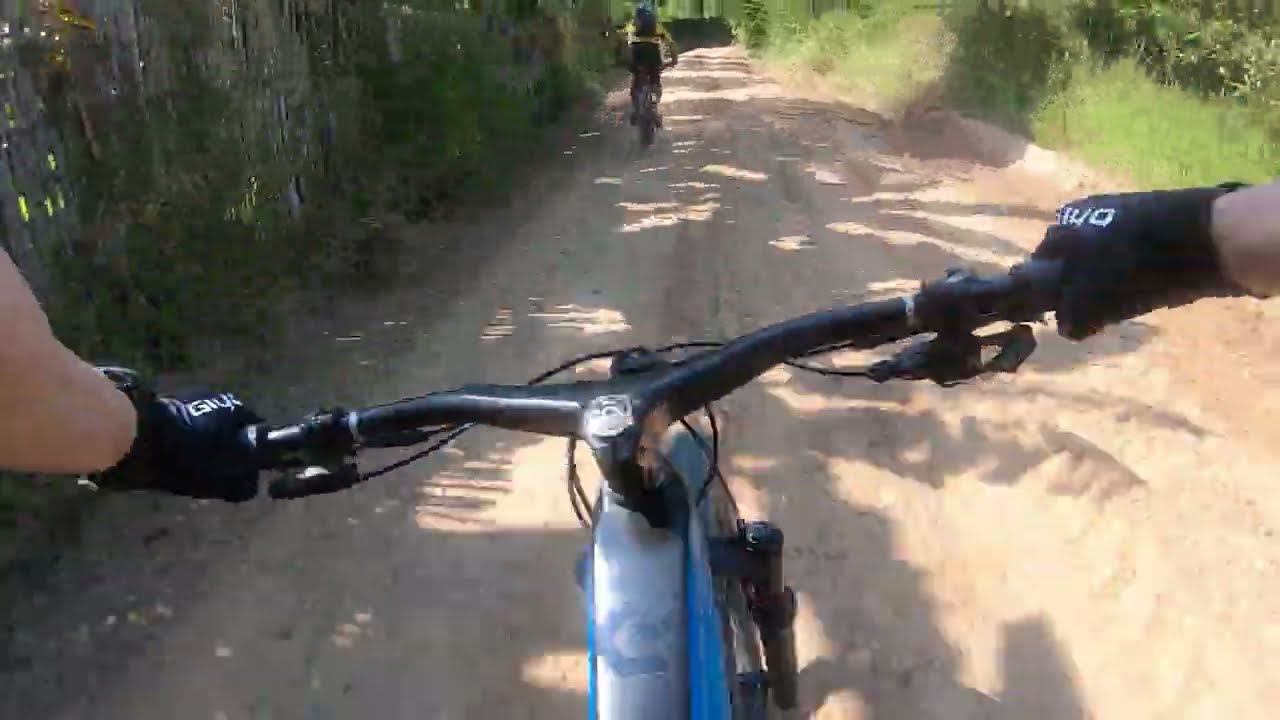The point-of-view image captures the exhilarating scene of a cyclist riding a silver and blue bicycle with black handlebars on a compacted sandy dirt road. The rider's hands, clad in black and white gloves, grip the handlebars firmly. Directly ahead, another cyclist on a black bicycle can be seen wearing a distinct yellow and black shirt featuring a silver reflective band across the center. The leading cyclist also dons black shorts and a backpack. The dirt road, tan in color, is flanked by vibrant green vegetation; the right side boasts shorter green grass interspersed with various bushes, while the left side is bordered by a row of trees forming a dense wall. Additionally, an old brown wooden fence with green vines climbing up it runs along the left side, allowing some light to seep through its gaps, casting shadows onto the trail. The path ahead curves slightly to the right, disappearing from view, inviting the riders onward.